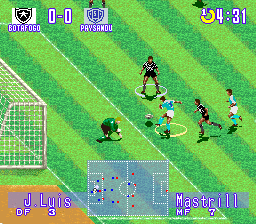This screen capture from a soccer video game showcases an intense match in progress. The field, illustrated with alternating striped shades of green grass, sets the stage for the action. Two teams are competing: one team is dressed in dark jerseys while the opposing team sports blue jerseys. Both teams’ players are also wearing matching shorts. Featured prominently are four players; two in dark shirts, and two in blue shirts. Nearby, a goalie, distinguishable by their green jersey, stands alert near the net, which is positioned to the left side of the image. 

At the bottom of the screen, a minimap provides an overview of the entire soccer field, while the player names "Jay Lewis" and "Mastril" are displayed for reference. Above, the game interface indicates a tied score of 0-0 and shows the elapsed time as 4:31. The immersive details capture the dynamic environment and competitive spirit of this digital soccer game.